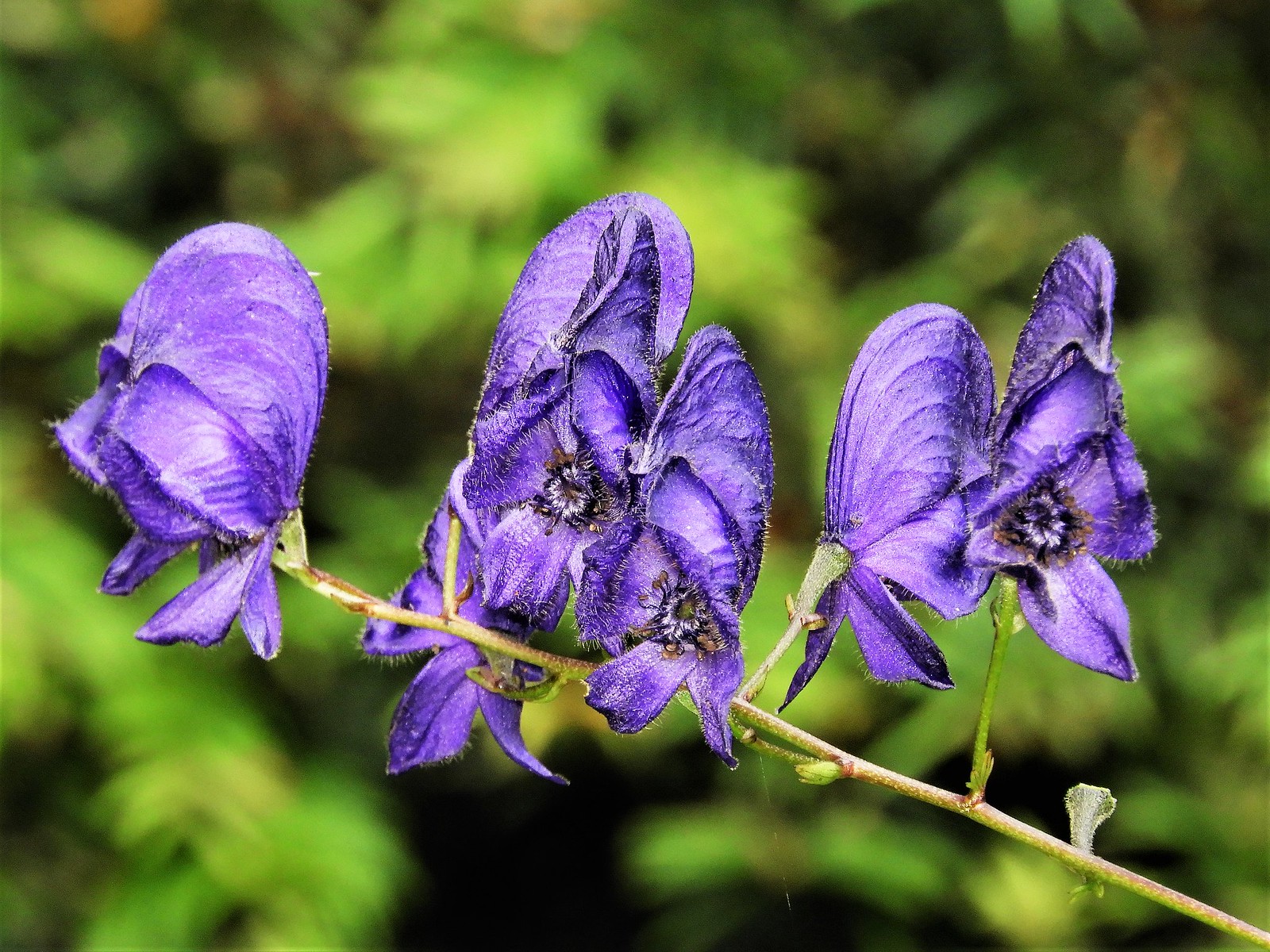This image, taken outdoors in daylight, features a close-up of a flowering plant. The main focus is a central stem that diagonally stretches from the bottom right to the upper left. The stem showcases a series of multiple purple buds, some of which are slightly open, revealing their inner white, black, and brown stamens. The five prominent bluish-purple flowers are interspersed with green buds that have yet to bloom. This floral specimen occupies roughly 80% of the central frame, making it the focal point. The background consists of blurred green vegetation with various highlights and shadows, evoking the presence of shrubbery and low bushes, possibly with a touch of yellow. The detailed texture of the flowers contrasts beautifully against the indistinct greenery, suggesting a natural, thriving outdoor setting.